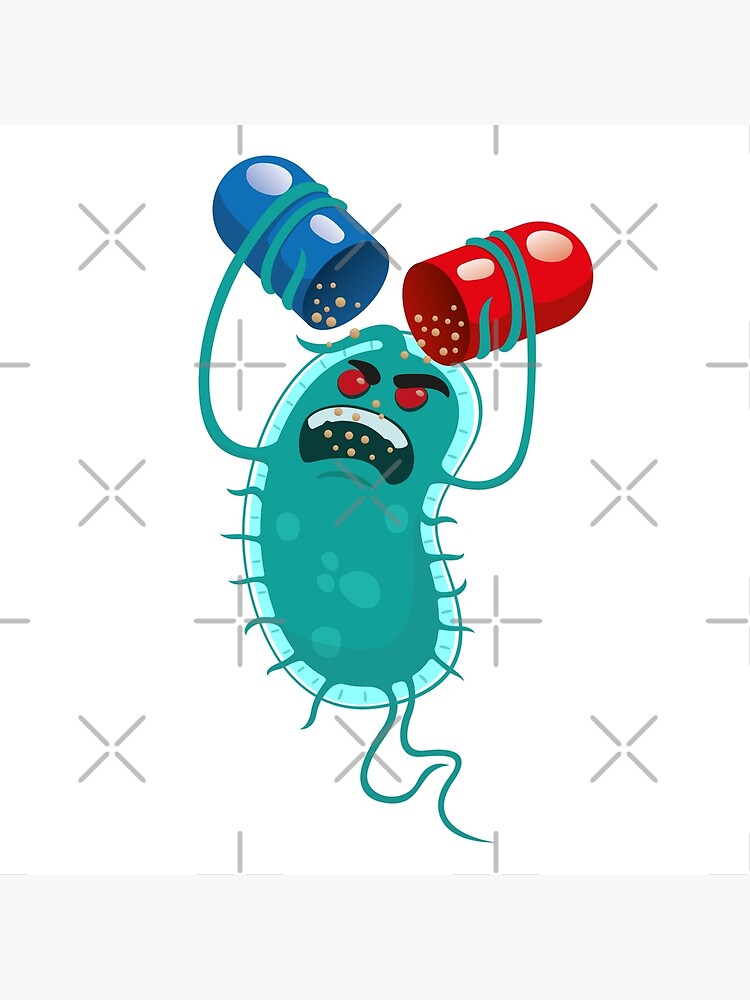This image is a digitally created graphic, likely sourced from a stock image library, evident from the grey grid lines overlaying the design and two horizontal grey lines framing the top and bottom. The central figure is an exaggerated, vibrant green creature resembling a bug or virus with numerous thin, leg-like appendages. The creature has a distinctly menacing appearance with its bright red eyes and expressive black eyebrows. It is characterized by two arms that are gripping a split medical pill, with the pill halves depicted in contrasting blue and red colors. From the pill emerges an array of small circular pieces that the creature appears to be ingesting. The combined elements create a cartoonish yet vivid representation, possibly symbolizing bacterial resistance to medication or illustrating a microbiome-related concept.